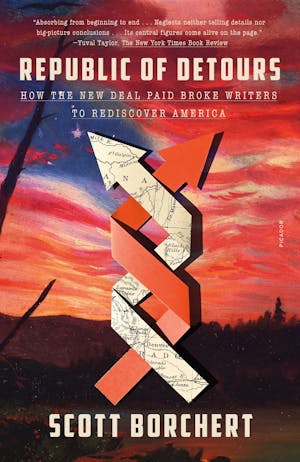This is a photograph of a book cover titled "Republic of Detours: How the New Deal Paid Broke Writers to Rediscover America" by Scott Borchert. The cover is predominantly red, white, and blue, with the sky artistically resembling the American flag. The sky features sweeping red and white streaks with a section of blue in the upper left corner. Central to the design are two intertwined arrows: one solid red pointing left, and another comprised of a map pointing right. Behind these intersecting arrows, a landscape of mountains and trees is visible. At the top of the cover, a quote from the New York Times Book Review describes the book as "absorbing from beginning to end."